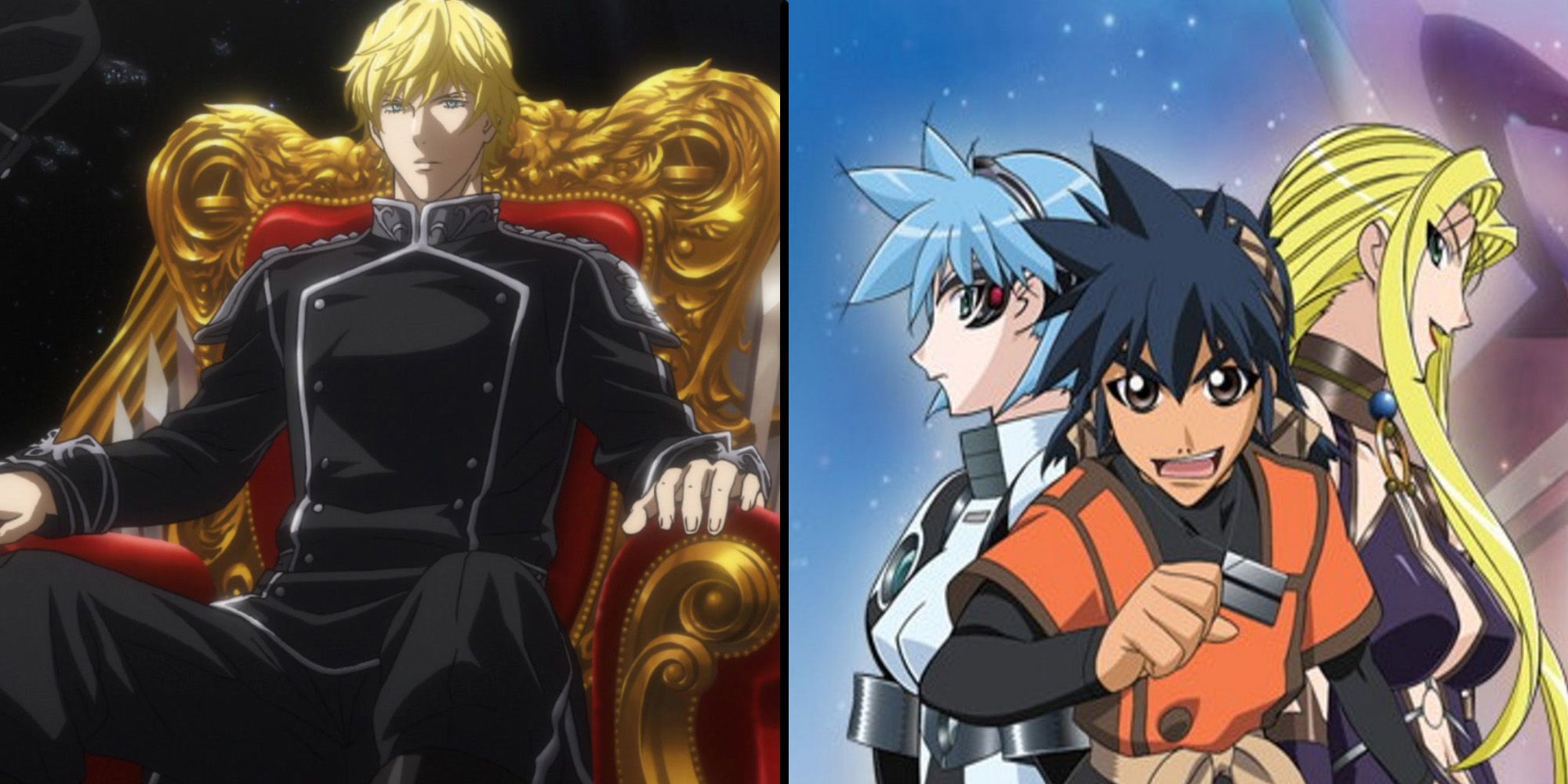The image is split into two panels, each showcasing distinct anime characters. On the left, a majestic, kingly figure is seated on a gold throne with deep crimson red cushions. This character, a white male with long blonde hair and blue eyes, is dressed in a highly detailed black military uniform adorned with silver linings and shoulder armor. His serene yet commanding presence is accentuated as he gazes outward, hands resting on the armrests.

On the right, three anime characters are presented. In the center stands a boy with spiky black hair, wearing an orange outfit with a long-sleeved black shirt underneath, his expression intense and dynamic. To his left is a woman with spiky blue hair, a black stripe under her left eye, and wearing a high-collared white suit that appears somewhat like armor. She also has a distinct black device near her eye with a red circle in it. To his right stands a woman with long blonde hair, dressed in a somewhat revealing dark purple or blue halter top with a cuff necklace. The background of this panel features shades of blue and purple, adding depth to the animated scene.